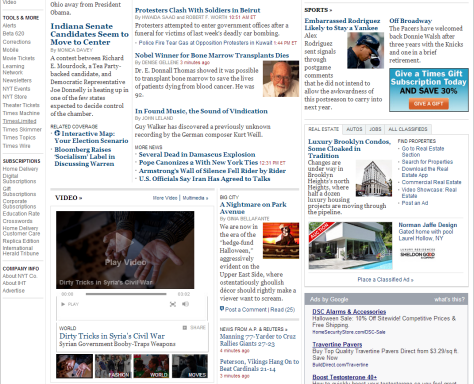A white, slightly blurry newspaper page heavily populated with text, prominently featuring black and blue sections. In black text, the words "Tools," "Move" or "Movie," "Alerts," "NYT," "New York Times Score," and subscription types including "Home Delivery," "Digital Subscriptions," "Gift Subscriptions," "Corporate," "Education," and "Crosswords" are visible. Further company information categories such as "About NYT," "Code About IHT," and potentially "Advertise" are also noted but less clear.

In blue text, headlines include:
- "Indiana Senate Candidates Seem to Move to Center"
- "Interactive Map: Your Election Scenario"
- "Bloomberg Races Socialism Label"
- "Discussing Warren"
- "Protests Clash with Soldiers in Beirut"
- "Nobel Winner for Bone Marrow Transplant Dies"
- "Found Music to Sound of Vindication"
- "Several Dead in Damascus Explosion"
- "Pope Canonizes With New York Tides"
- "Enron's Wall of Silence Fell Writer by Writer"
- "U.S. Official Says Iran Has Agreed to Talks"
- "Nightmare on Park Avenue"
- "Dirty Tricks in Syria's Civil War"